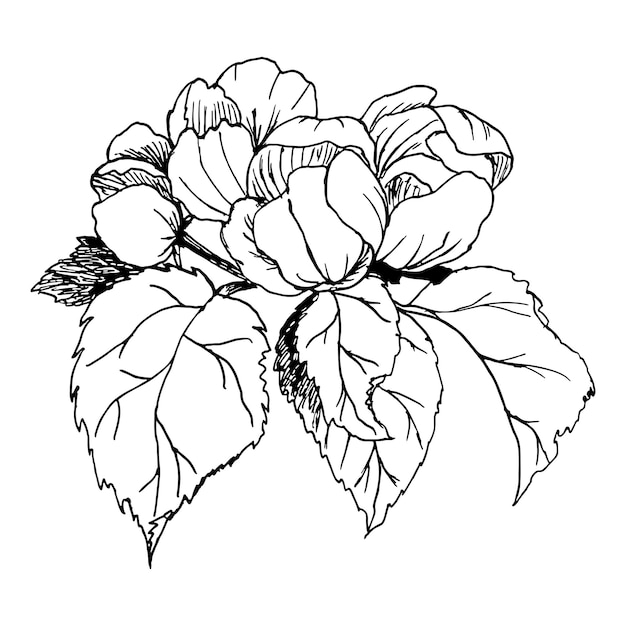This intricate black and white drawing, rendered in black ink, showcases a bundle of flowers and leaves. At the top, there are several flowers—likely peonies or possibly magnolias or gardenias—with a mix of open and partially open blooms. The left side prominently features three buds that have yet to open. Below the flowers, there is a detailed arrangement of large leaves, four in total, each exhibiting distinct characteristics. The largest leaf is on the left, with a smaller leaf positioned in the middle, accompanied by another in front with a jagged, darker edge. The right side displays a leaf that faces outward. The drawing also includes veins on the leaves and shading applied with careful precision, adding depth and dimension to this monochromatic artwork set against a white background.